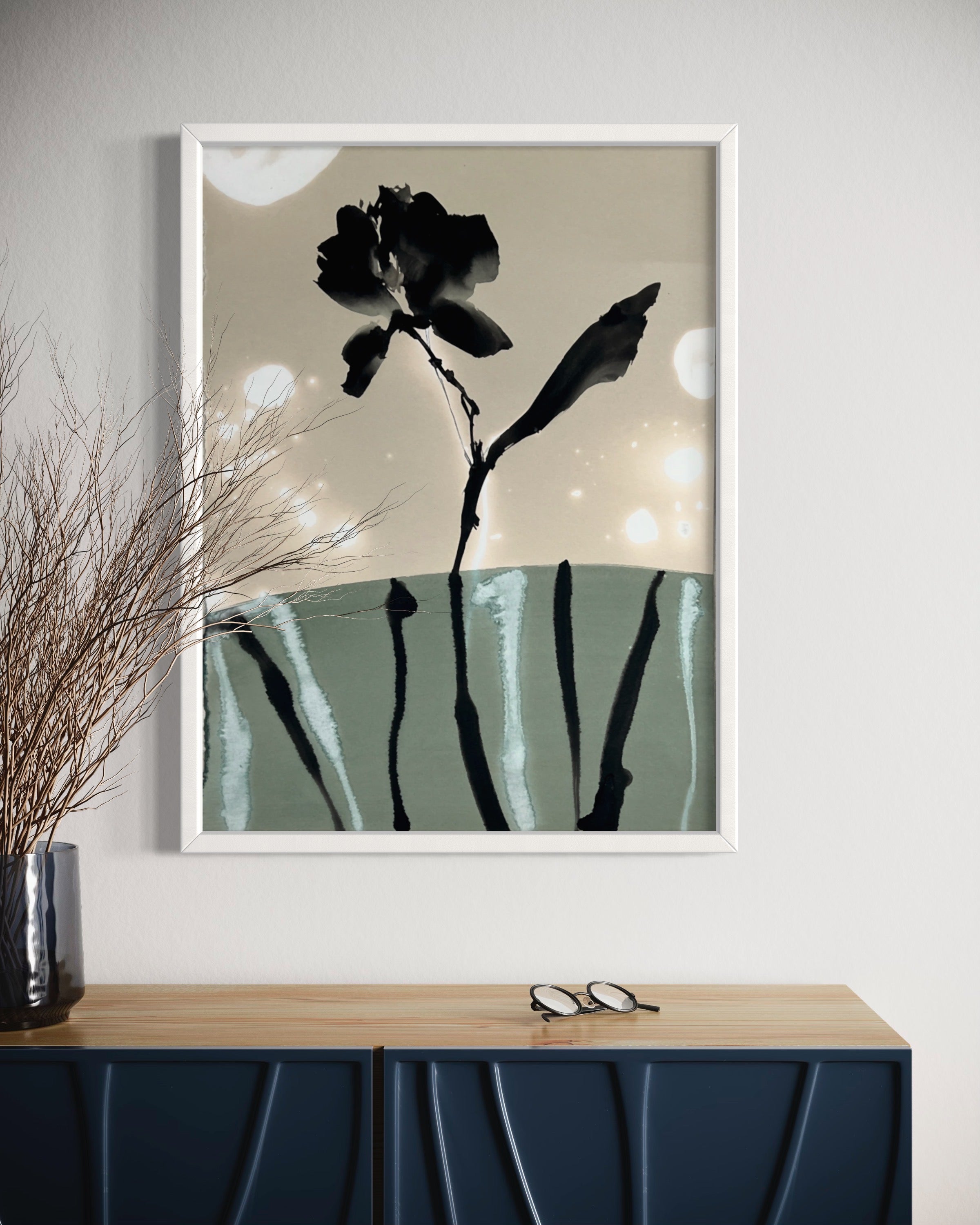The image is a detailed photograph taken indoors, showing a well-organized setting. Central to the composition is a stylish cabinet with a brown wooden countertop and contrasting gray doors. Resting atop this cabinet is a pair of black, round-framed glasses and a sleek, silver vase containing dry brown plants. The backdrop features a white wall adorned with a vertically oriented, rectangular framed artwork. This artwork depicts an iris plant in silhouette against a gray sky with white spots, complemented by adjacent branches. The painting incorporates subtle hues of green within its predominantly black, gray, and white palette and is bordered by a white frame. The scene exudes a balanced, aesthetic juxtaposition of natural elements and clean, modern design.